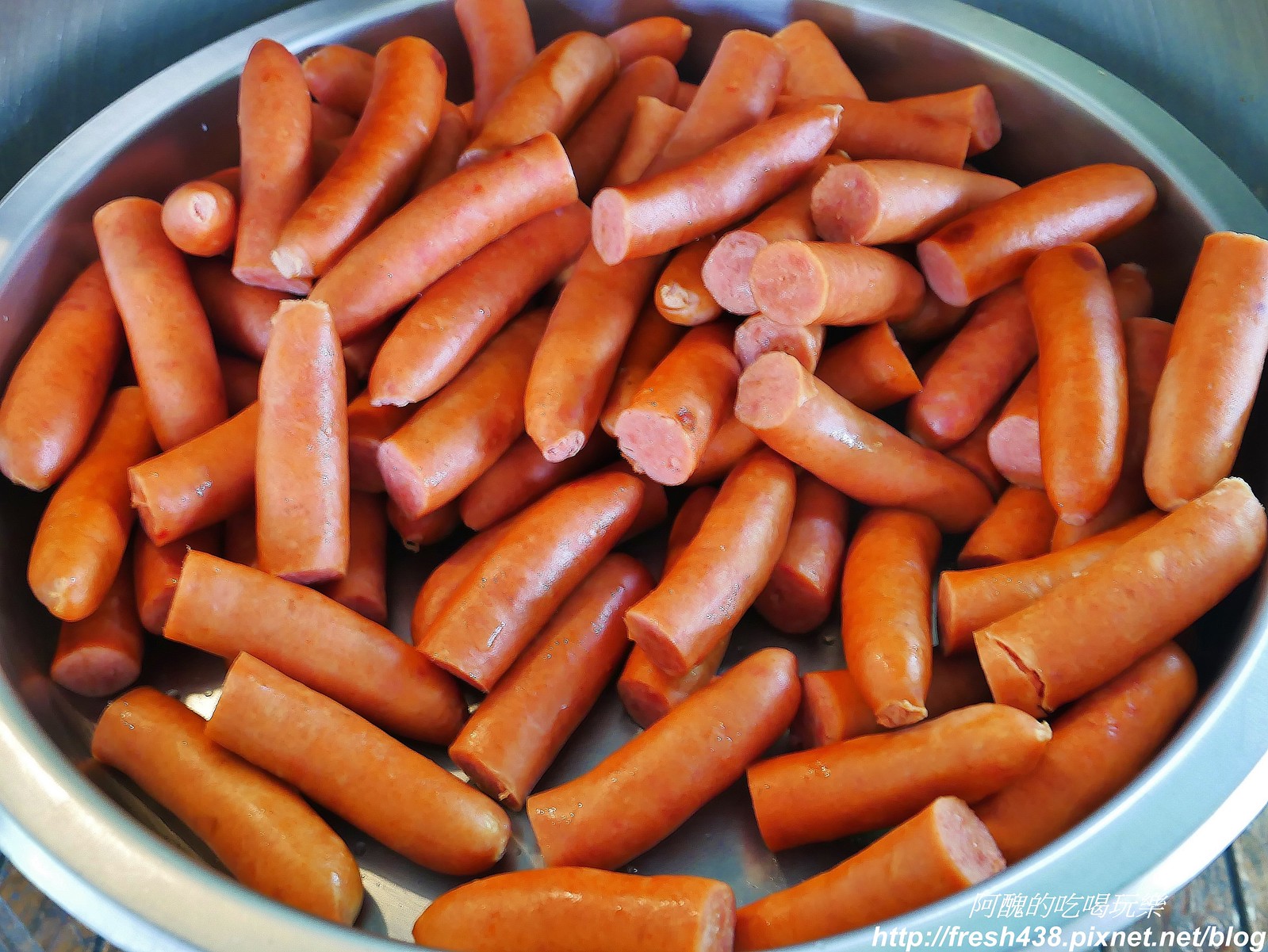The close-up photograph depicts a large quantity of cut-up sausages or possibly Vienna sausages, resembling hot dogs, filling a shallow, metallic blue-tinted circular bowl that looks similar to a pie pan. The sausages, approximately 40 to 60 in number, are evenly halved, showcasing an outer skin with a reddish-brown hue and a lighter pinkish inner meat, indicative of pork. Each cut end forms a flat circle, highlighting the texture and color contrast between the outside and inside of the sausages. The background surface is barely visible but might be grey or wooden, and the photograph includes a URL at the bottom right corner in white text, partially accompanied by Asian characters, reading "http://fresh438.pixnet.net/blog."